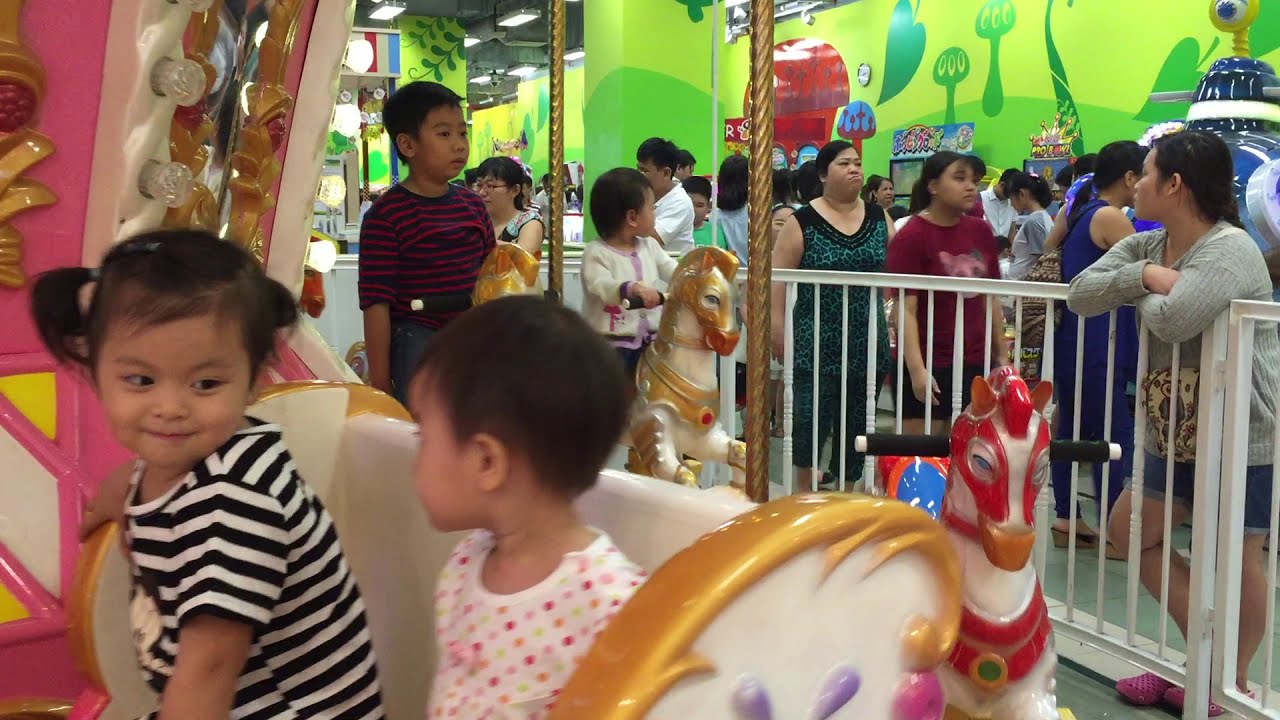The image captures a lively scene at a carnival, with two young children, around three years old, prominently featured in the foreground. They are seated together on a shiny white and gold bench of a merry-go-round. One child, likely a girl, has dark hair styled in pigtails and wears a black and white striped shirt. The other child, also with dark hair, sports a white shirt adorned with pink and green polka dots. They look at each other, sharing an intimate moment amidst the excitement.

Surrounding them on the ride, several other children can be seen, including one standing and another sitting on the classic merry-go-round horses with gold trimmings. The ride is bustling with activity.

Beyond the merry-go-round, a metal gate keeps additional visitors at bay, while a line of people, including various adults and children, waits expectantly. Among the crowd, notable figures include a woman in a gray sweater and blue shorts watching the children, and another in a red t-shirt near an older woman in a green dress. These individuals add to the vibrant, busy atmosphere of the scene.

The background features green walls decorated with colorful drawings of trees, contributing to the playful and whimsical environment. Overhead, fluorescent lights illuminate the setting, highlighting the vivid details and making it clear this is a place bustling with joyful activity. The combination of the engaging background, the lively crowd, and the charming interaction between the children captures the essence of a fun-filled day at the carnival.